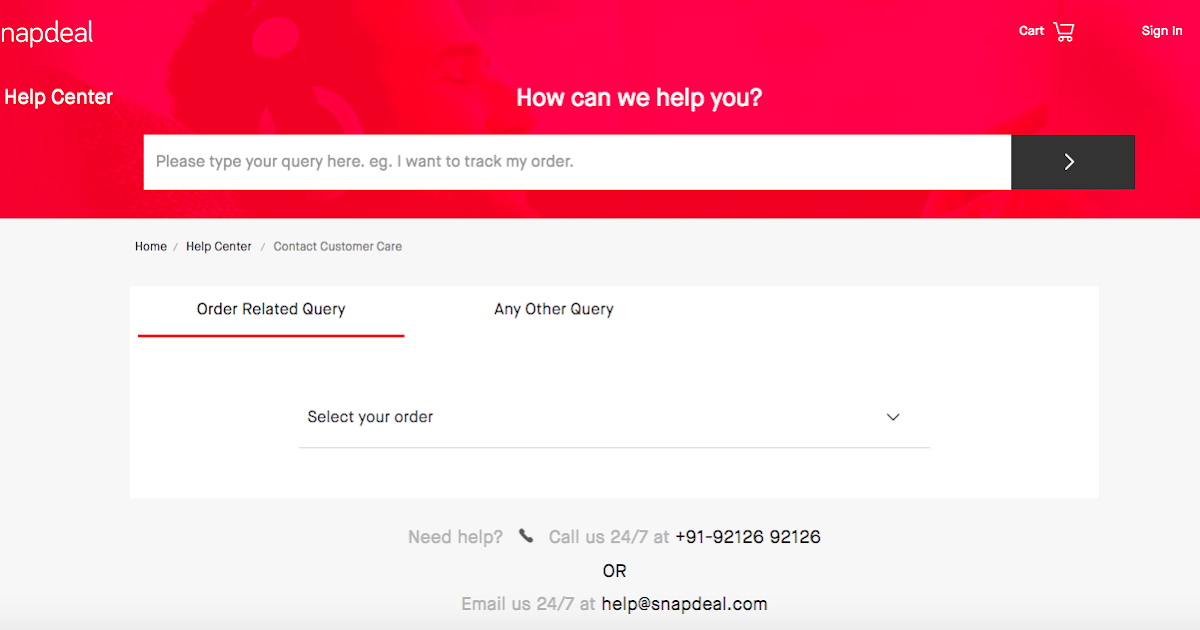This image depicts a section of the Snapdeal website, specifically its Help Center page. In the top-left corner, a partially visible "Napdeal" is seen due to the cut-off, with the missing 'S' confirming it as Snapdeal. The header area is dominated by a red background which features the image of a man wearing headphones, suggesting customer support. The header includes various useful icons and buttons, such as the cart button, "Sign In," and the Help Center link, all in white text.

The central portion of the page displays a search bar under a helpful prompt that reads, "How can we help you?" Users are encouraged to type their queries into the search bar, which contains a placeholder text saying, "please type your query here." Beneath this, there is an example query, "I want to track my order," and a black search button to the right allows users to finalize their search.

Further down the page, navigation options are clearly labeled: "Home," "Help Center," and "Contact Customer Care." The "Order Related Query" section is currently highlighted, indicating its active status. An additional section for "Any Other Query" is also available, alongside a dropdown menu labeled "Select your order," which is set to "Everything" at the moment. 

Towards the bottom of the page, there's a gray text section asking, "Need help?" followed by a phone icon. The text provides a 24-7 customer support contact number: "+91-92126-92126," and an email address for assistance: "help@snapdeal.com." This contact information, along with the format of the phone number, suggests that the website operates outside of the U.S., likely in India.